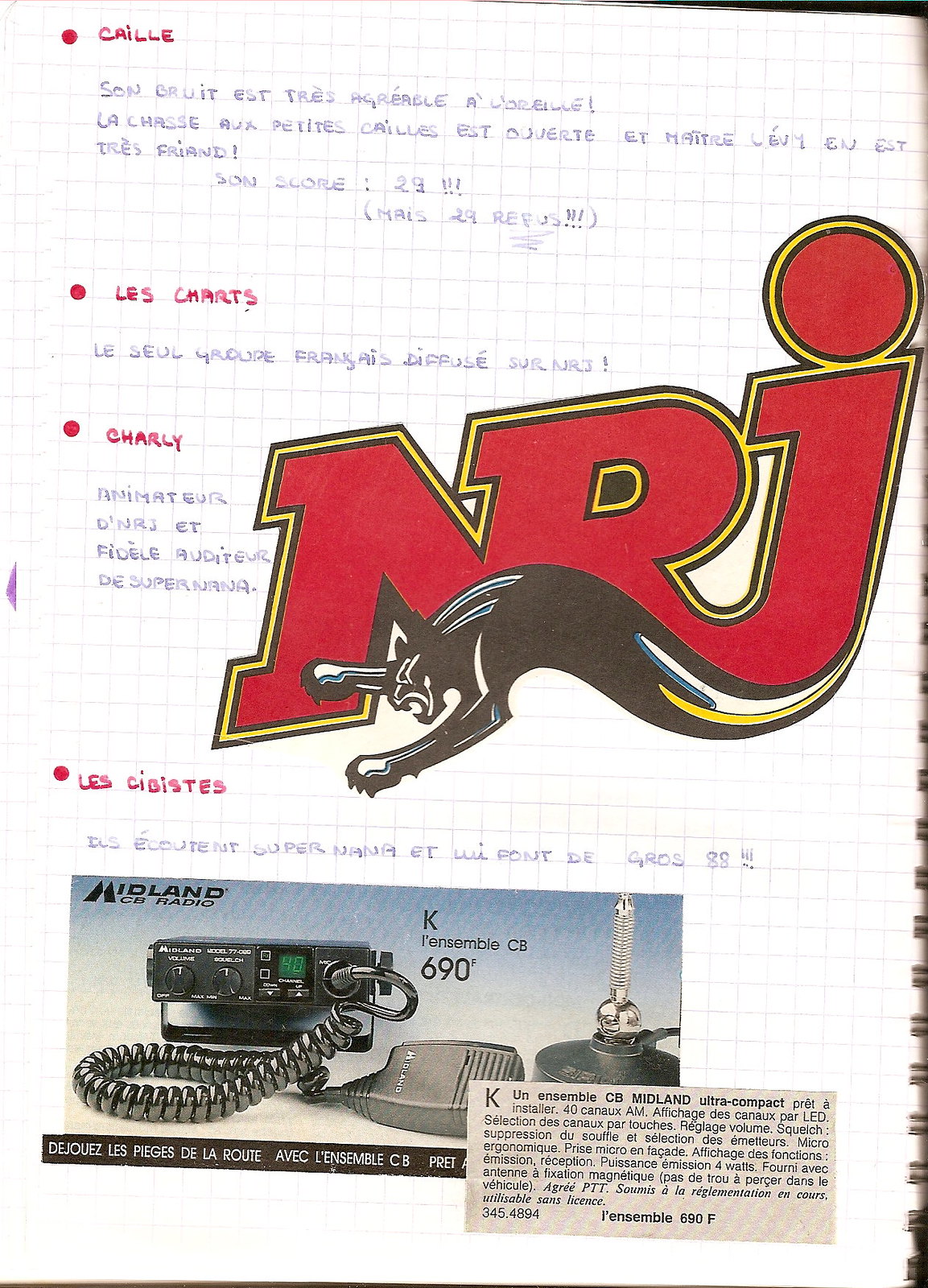The image is a close-up digital scan of a page, likely from a spiral-bound notebook, identifiable by the binding visible on the right side. The page appears to be a photocopy or a graph paper with vertical and horizontal lines, and is filled with text mostly in French. At the top, there are four bullet points written in red, which read: "C-A-I-L-L-E," "L-E-S-C-H-A-R-T-S," "C-H-A-R-L-Y," and "L-E-S C-I-B-I-S-T-E-S." Prominently featured in the center of the page is a large "NRJ" logo, with a panther emerging from the bottom of the "J." At the bottom of the page, there is a detailed advertisement for a CB radio, specifically featuring Midland CD Radio models. The description includes terms like "K Ensemble CB 690F," "K Ensemble CD Midland Ultra Compact," and possibly mentions something related to "Installer 40 Canux AM." The overall layout and content suggest the page is an informative flyer or promotional material featuring both written details and a photograph of the electronic device.